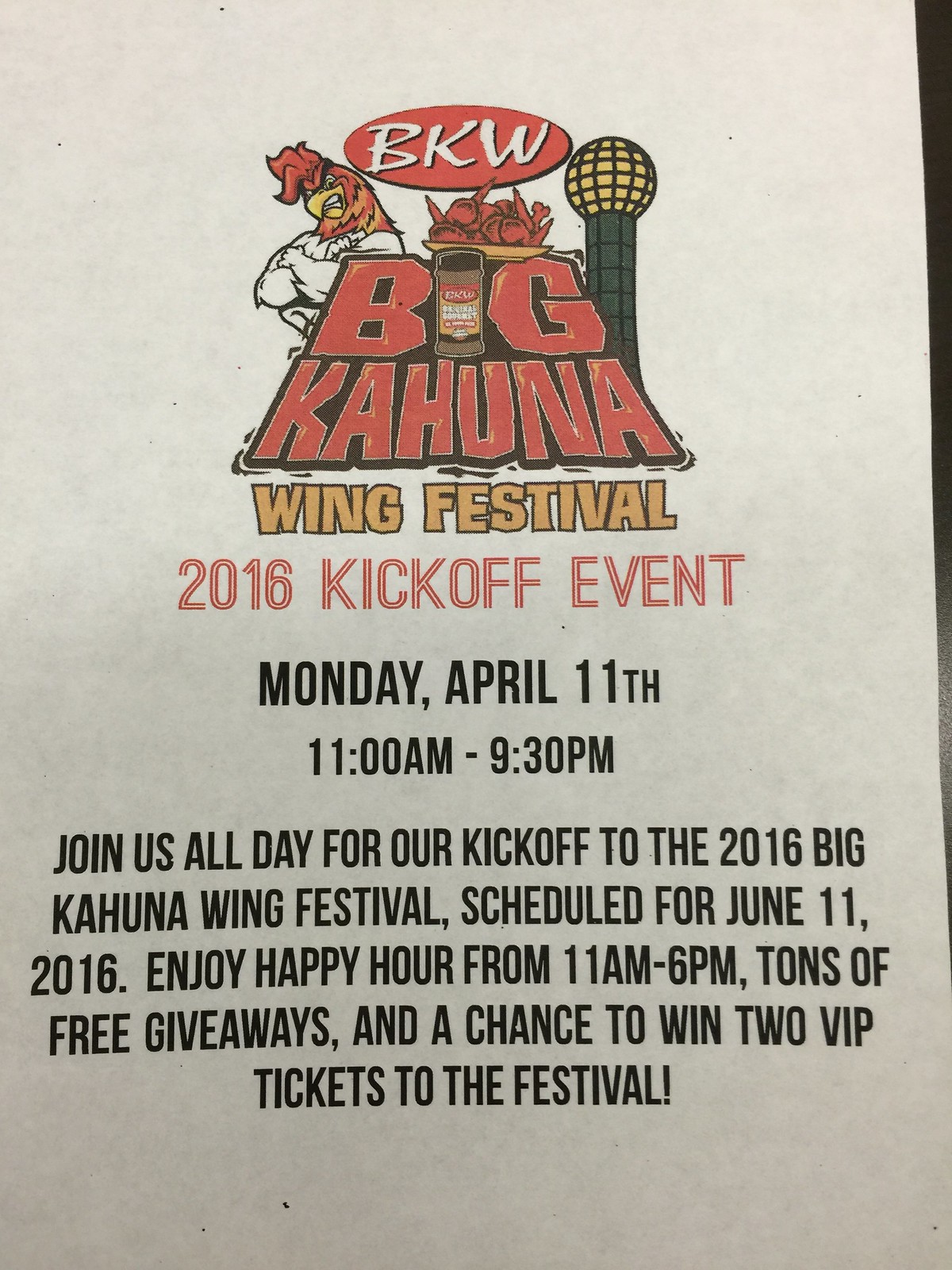The image is an advertisement featuring a poster for the Big Kahuna Wing Festival 2016 kickoff event. The poster has a white background with vibrant and varied lettering. At the top, the letters "BKW" are encased in a red oval. Below that, the "Big Kahuna" text is prominently displayed in large red letters where the "I" in "Big" is stylized to look like a seasoning container. This is followed by "Wing Festival" in bold, yellow letters. 

A central figure on the poster is a muscular chicken or rooster with a white body, brown head, yellow beak, and a red comb, standing with scowling face and folded arms. To its right is a plate of cooked wings and a tall, cylindrical microphone with a globe on top. The details of the event are clearly listed underneath: 

"2016 Kickoff Event, Monday, April 11th, 11 a.m. to 9:30 p.m." The message continues in black text, inviting guests to join the kickoff festivities for the June 11th festival. Highlights include happy hour from 11 a.m. to 6 p.m., free giveaways, and a chance to win two VIP tickets to the main event.